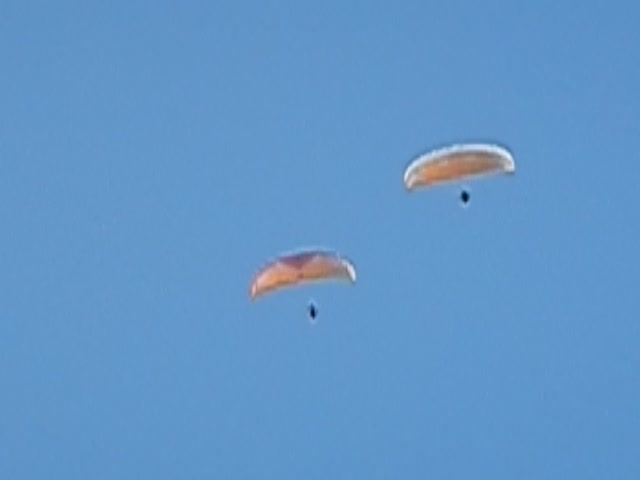In this daytime photograph taken from the ground, you can see two distant figures that resemble tiny black dots, indicating their considerable height in the sky. Both individuals are parachuting under wide canopies. The parachutes are described as an off-white color, though one has a possible red triangle marking. The sky is a clear, uninterrupted blue without any clouds or other objects. The parachutists are relatively close to each other, with the one on the bottom left slightly lower than the one on the right. Despite the image's blurriness and the extreme distance, it captures the descent of these skydivers against the expansive blue sky.